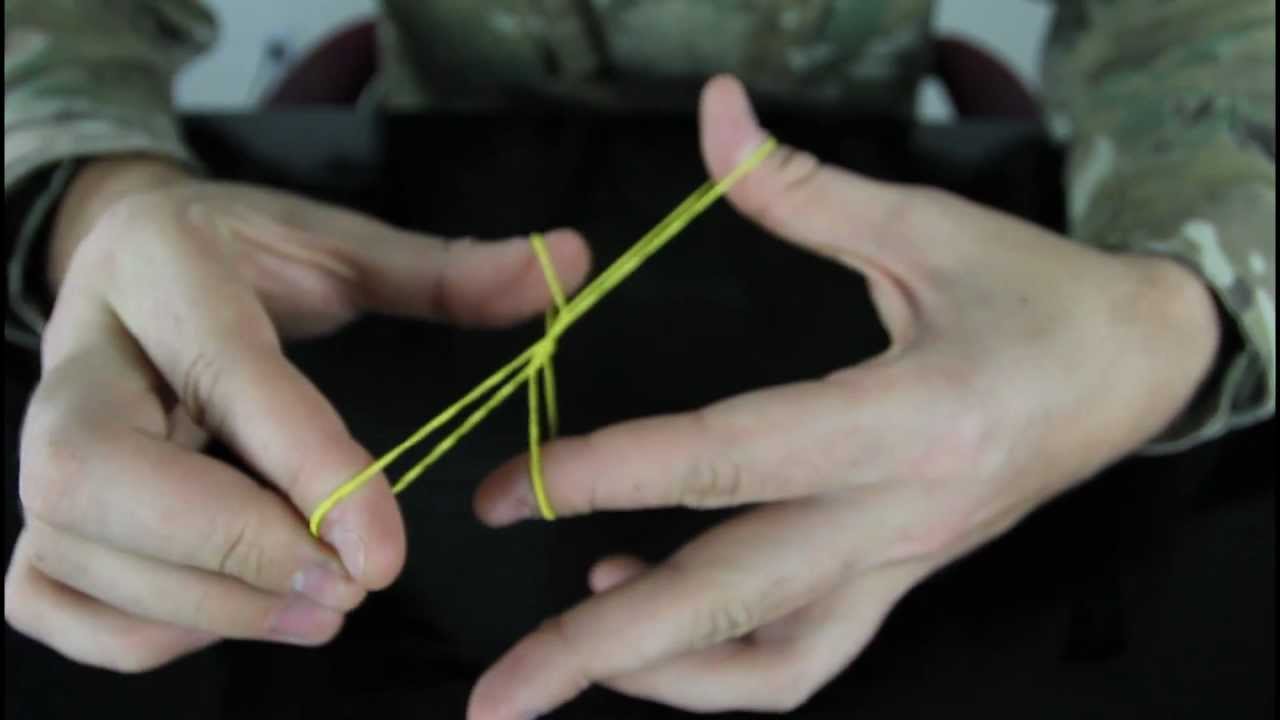In this detailed close-up image, two hands, presumably belonging to a Caucasian person, are manipulating yellow elastic bands in a complex, intertwined manner over a shiny black table. The hands are contorted in a distinctive shape typical of individuals knotting or performing tricks with string or rubber bands. Each hand has the elastic bands wrapped around the thumbs and forefingers, forming an "X" pattern between them. The person is dressed in long-sleeved camouflage military fatigues, indicating possible army apparel, with a background that is predominantly white. Only a small portion of the person's upper body, including parts of the arms and chest, is visible, suggesting they are seated closely to the table.